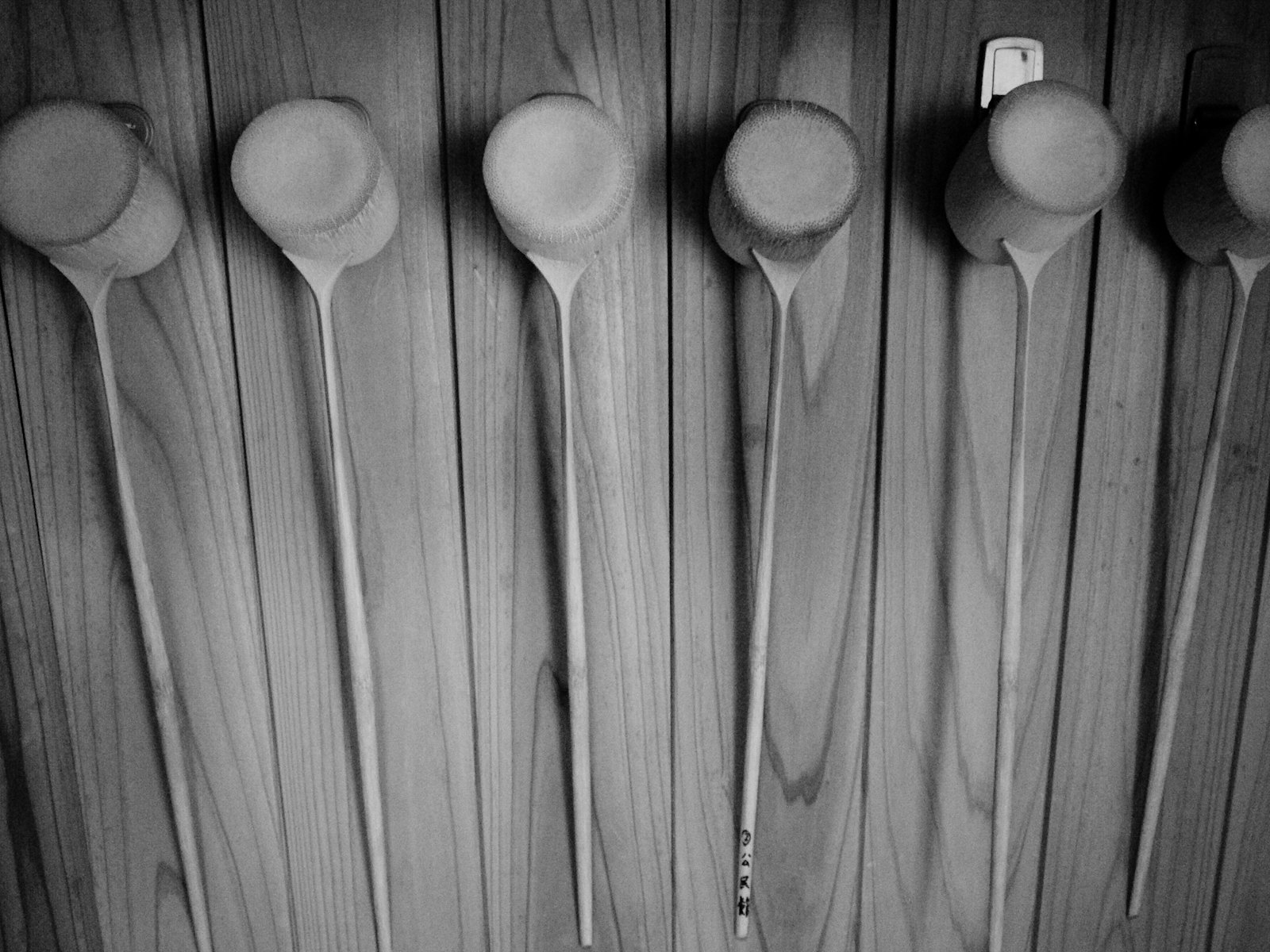In this black-and-white photograph, there are six tall, slender wooden ladles mounted on a wood-paneled wall. Each ladle consists of a shot glass-sized cylindrical bowl attached to a long, thin handle. The bowls, which resemble small wooden pegs or cups, are affixed to the wall with silvery hooks, resting edge-down against the vertical wooden panels. Notably, the fourth ladle from the left features black symbols resembling Chinese characters on its bowl, while the others are unmarked. The wooden grain and texture are prominent, suggesting a bamboo-like material. The composition gives an impression of a set of purposefully arranged traditional utensils.